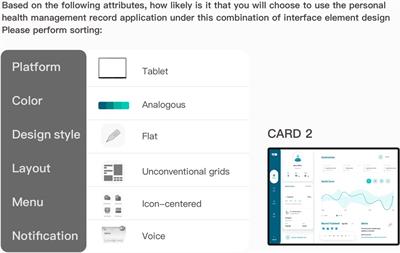This image is a detailed screenshot from a survey regarding a personal health management record application. At the top, the question posed is, "Based on the following attributes, how likely is it that you will choose to use the personal health management record application under this combination of interface element design? Please perform sorting." The left column lists various attributes for sorting, including platform, color, design style, layout, menu, and notification. In the middle, there are icons representing different choices such as a tablet for platform, analogous for color scheme, a pin icon labeled flat for design style, unconventional grids for layout, icon centered for menu configuration, and voice for notifications. At the bottom right, there's a sample card labeled "Card 2" presumably illustrating a preview based on the selections made. The purpose of the image is to allow users to sort and match various interface elements to personalize the application design.